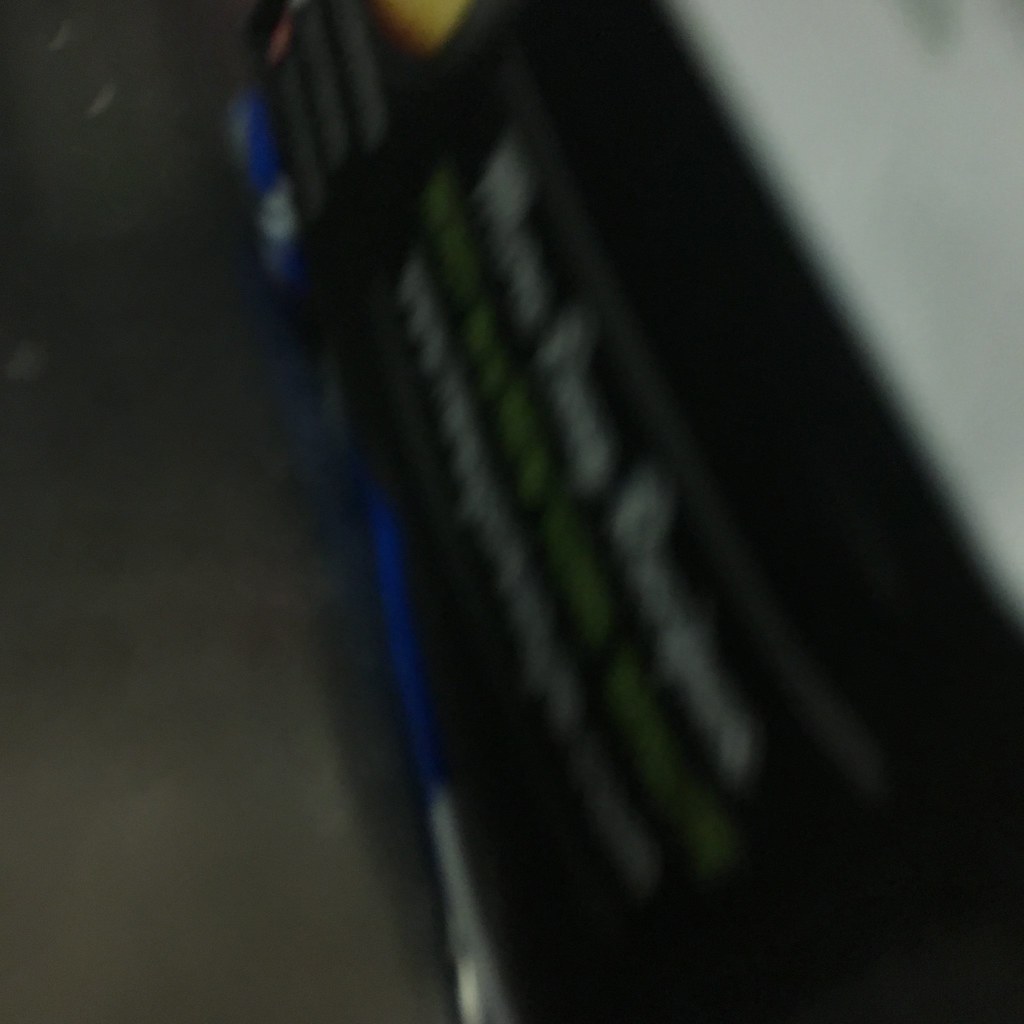This image is an extremely blurry photograph with indistinguishable details, making it challenging to decipher. The scene seems to be taken from an elevated perspective, possibly looking down at a dark, concrete-like floor or road on the left side, which is a medium to dark gray. Centered in the image, there is a prominent large black object that might be the size of a car bumper, featuring multiple lines of text—white on the top line, green in the middle, and white again on the bottom—but the text is unreadable due to the blur. Above this large black item is another section of black with some smaller black lines, and topping it off is a white patch. Below the main black object, there appears to be a silver and blue pole-like feature, potentially a broom. The placement and environment suggest it might be a warehouse or garage setting.